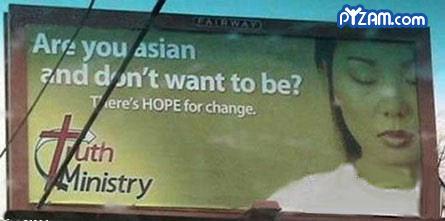The image showcases a billboard with a prominent, detailed design. The background of the image is a light blue gradient, most noticeable around the top and to the right. In the upper right corner, there's a URL that reads "PyZam."

The billboard itself features a red border and the word "Fairway" prominently displayed at the top section. The background color of the billboard is a greenish hue. In the central part of the billboard, a controversial message in white lettering reads, "Are you Asian and don't want to be? There's hope for change."

On the lower left of the billboard, the word "Truth" is written in red, followed by "Ministry" in black letters below it. To the right side of the billboard, there's an image of an Asian woman with her eyes closed, dressed in a white shirt. The overall composition blends multiple colors and textual elements intended to capture attention.